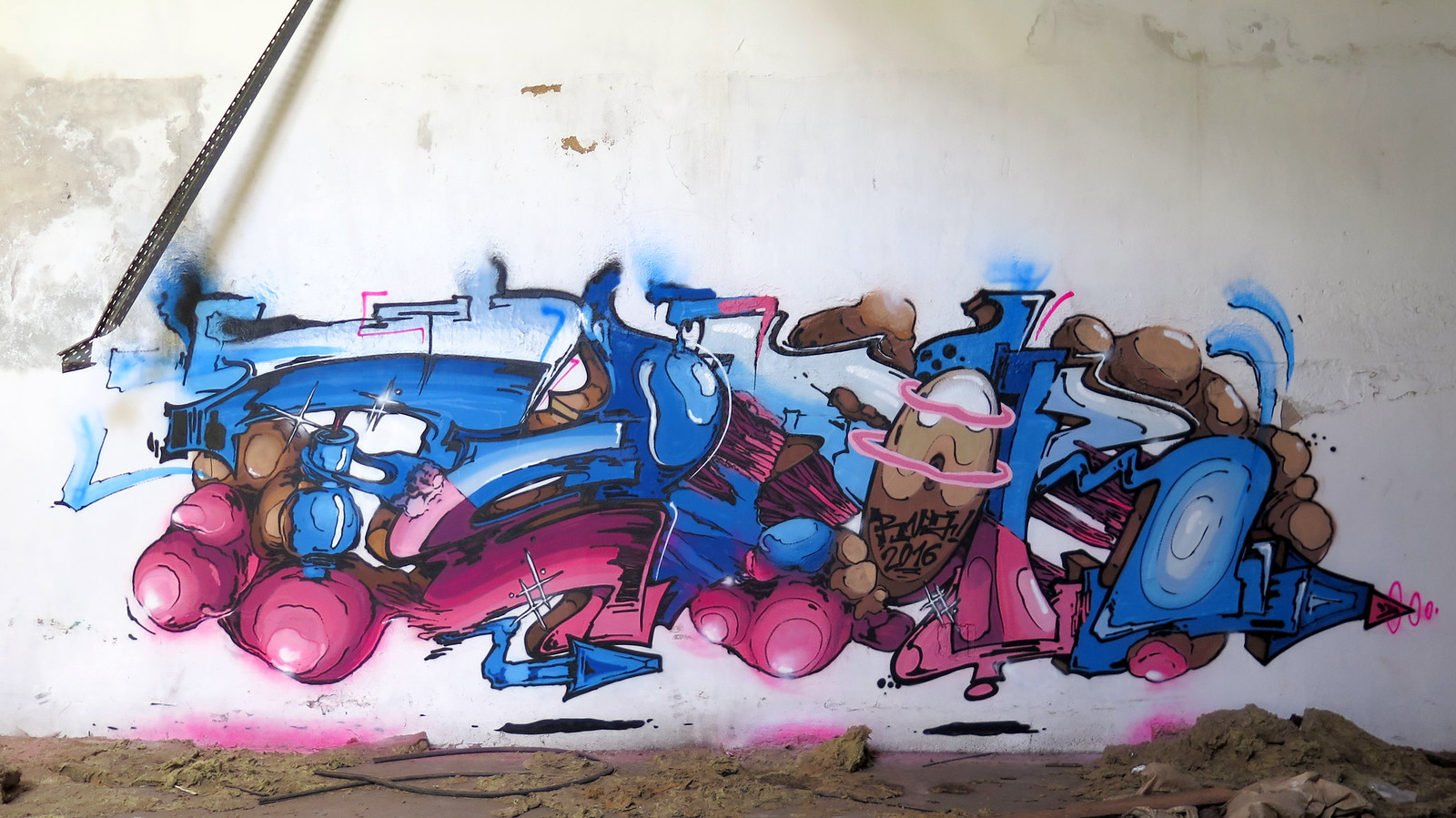The image depicts an outdoor scene featuring an abstract piece of graffiti prominently displayed on a weathered white wall, which appears to be under an overhang or bridge due to the interplay of light and shadows. The wall shows visible signs of wear with areas of chipped paint, exposing brown patches, notably on the left side and upper right corner. The ground in front of the wall resembles sandy terrain dotted with brown, dirt-like spots, and a rope or circular wire lies across it. 

The graffiti itself is a vibrant mix of colors predominantly featuring shades of pink, fuchsia, light blue, dark blue, white, and brown. Central elements include a large pink circular shape at the bottom, which has round, pink, donut-like features with a black unreadable tag resembling a donut with white icing on one tip. Above this are various blue hues forming abstract shapes, including a distinct blue arrow pointing to the right. There is also a brown oval shape encircled by pink rings, suggestive of an egg, near the top right. Another arrow, this time with blue coloration, emerges from the bottom of the graffiti. Small sections exhibit what looks like brown smoke and additional round, circular elements contributing to the abstract theme. 

On the far right, attached to the wall but separate from the graffiti, hangs a real wire that casts a shadow, adding depth to the photo. The scattered elements and vibrant colors of the graffiti create a visually intricate and abstract composition that resists easy interpretation.